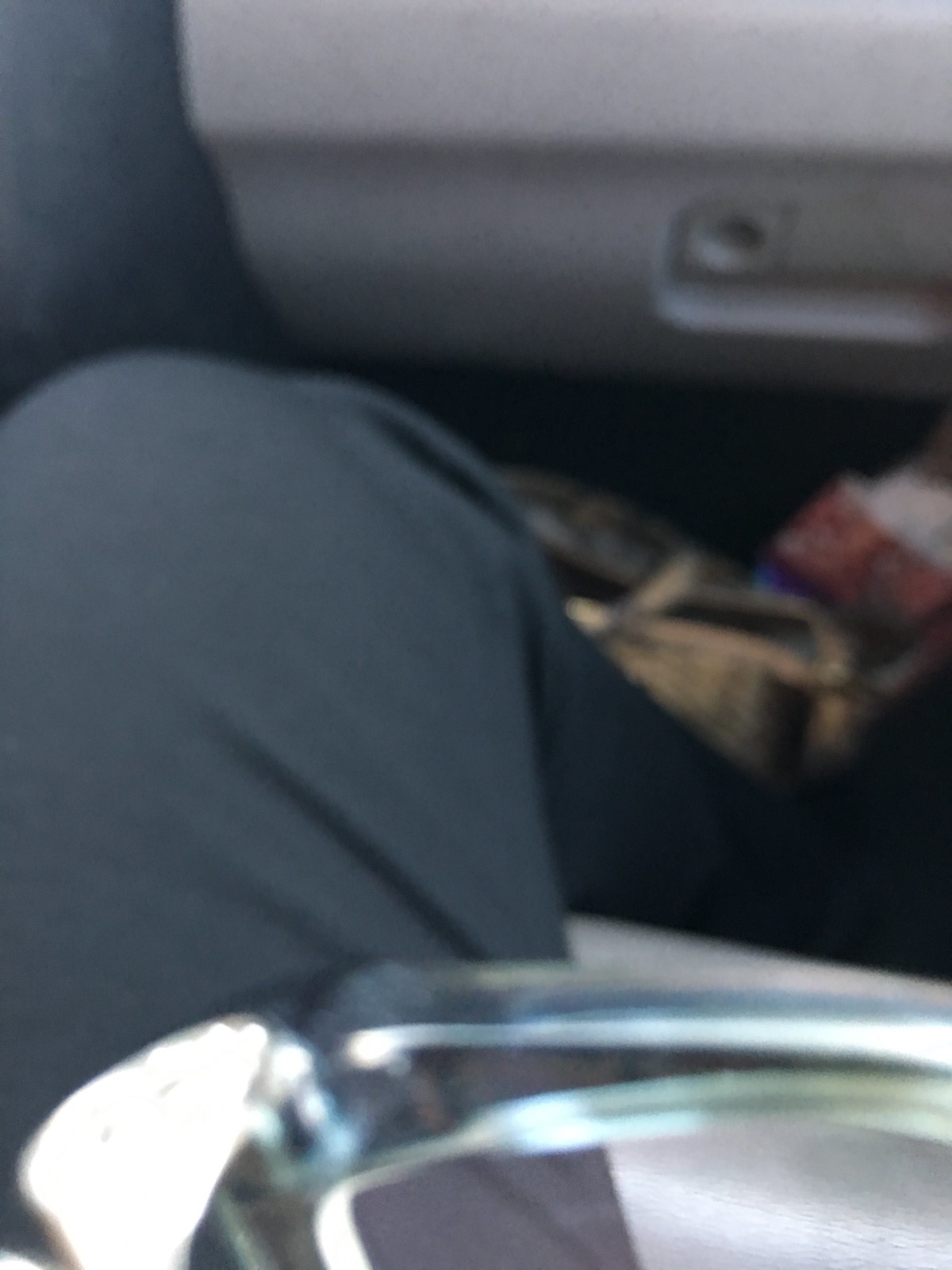The image depicts the passenger side of a car, highlighting various interior elements. In the foreground, the light gray dashboard extends seamlessly into a darker gray segment, identified as the glove compartment. The compartment door is ajar, offering a glimpse into an organized space for storage. On the floorboard beneath, an open bag reveals a mix of colorful items with hints of white, red, blue, and green peeking out from within. A person's leg, clad in dark gray pants, is prominently visible, with their shoe resting on the car floor. The individual appears to be wearing a gray and silver jacket, adding to the monochromatic theme of the scene. A slightly blurry white object, potentially a metal buckle, floats indistinctly in the composition, adding a mysterious element to the image. The overall photograph offers a snapshot of the vehicle's interior, captured with a focus on both the inanimate objects and the partial human presence.